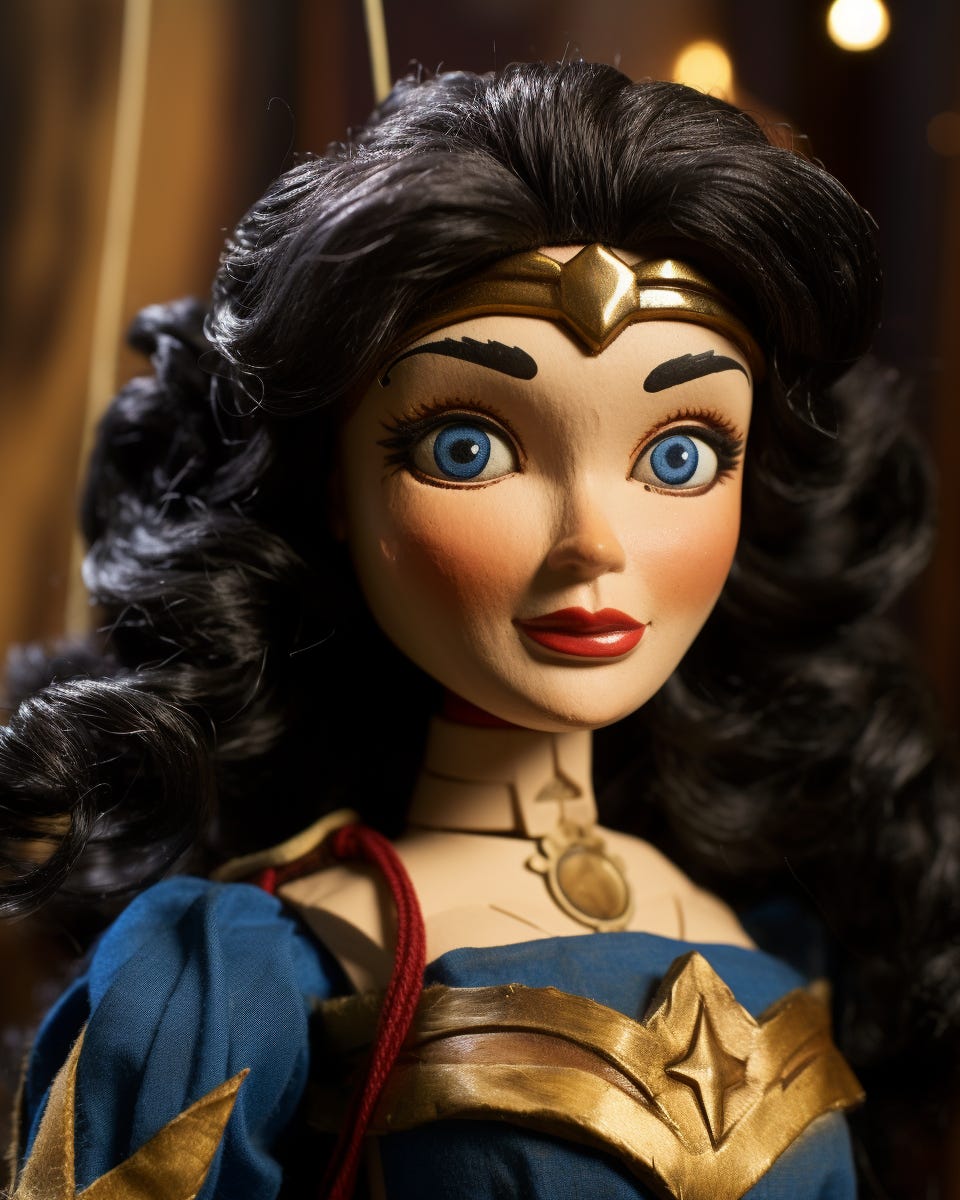This is a detailed photograph of a Wonder Woman doll, characterized by her long, wavy, and intricately curled black hair. She wears a distinctive golden headband, known as a tiara, adorning her forehead and complementing her thick dark eyebrows. Her facial features are meticulously crafted, showcasing big blue eyes with intricate highlights, well-defined eyelashes, rosy pink cheeks, and bold red lipstick. Around her neck, she wears a necklace adorned with a small gold charm.

The doll is dressed in a blue outfit with a prominent golden chest plate featuring a design similar to the golden emblem on her tiara. A touch of gold also embellishes the upper part of her sleeve on her right arm. Additionally, there appears to be a red lasso draped over one of her shoulders, hinting at Wonder Woman's classic accessory. The photograph is cropped at the breastplate, leaving the lower portion of the doll out of view. The background of the image is a blurred, uniform golden hue, adding a dramatic focus on the doll without any discernible elements behind her.